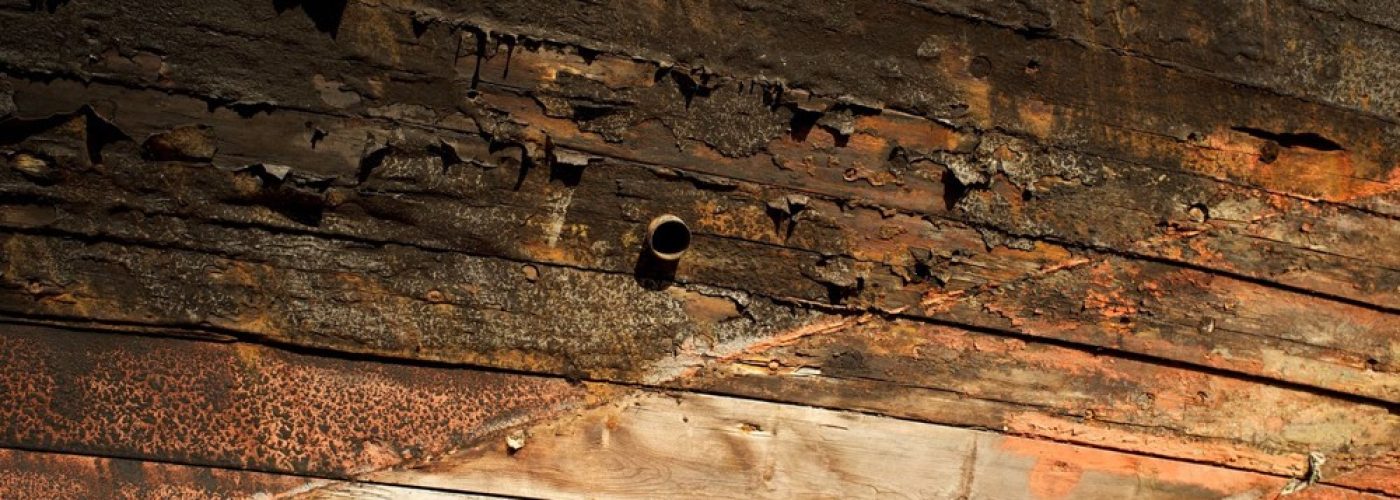This color photograph features a close-up view of several wooden planks, possibly remnants of a table or deck, displaying varying degrees of damage. The wood appears to have been affected by fire, evidenced by the seared, dark brown, and blackened sections, while some areas show peeling paint, contributing to the deteriorated look. The image reveals a gradient of destruction from top to bottom: the upper sections are severely blackened and flaking, suggesting intense burning, while the lower sections, particularly on the right, exhibit lighter damage, with patches of exposed natural wood and minimal scorching. A shiny board towards the bottom may have partly escaped the fire's wrath. At the center of the photograph, a mysterious metal ring rests on the planks, indicating either an integrated pipe or an inadvertent object. The overall appearance of the planks shows a transition from bright orange and brown hues on the right to dark, muddy tones on the left, marked by spots of mold and signs of long-term decay.